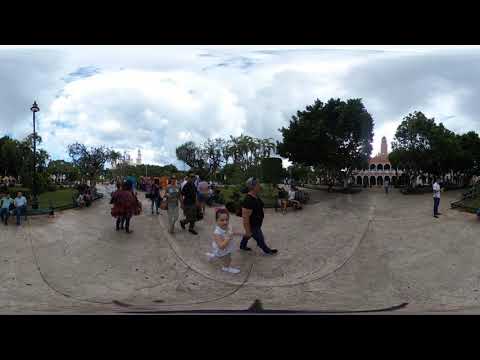This panoramic photograph captures an outdoor scene dominated by a central cobblestone pathway, subtly curved due to the panoramic distortion but likely straight in reality. In the middle, a little girl, seemingly enjoying an ice cream cone, holds hands with her tattooed father, who is in a t-shirt and boots. The backdrop displays a picturesque environment: an intricate old Byzantine building with grand archways, likely a tourist attraction. The area is adorned with well-maintained greenery, including trees, bushes, and garden beds. Puffy white clouds fill the light blue sky above. Approximately 16 to 20 people, dressed warmly, are sparsely dispersed along the pathway, giving a sense of liveliness. On the right side of the image, nestled among the trees, stands a large two-story building, potentially a museum or church, along with a tall light pole and an additional building peeking from behind the foliage. The entire setting suggests a well-visited park or historical site.